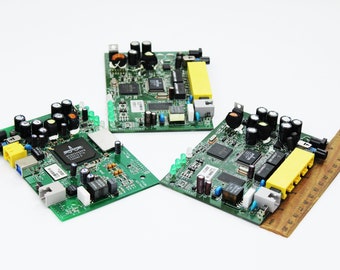The image depicts three unmounted computer motherboards laid out on a light gray or white background. These motherboards, small in size, display various intricate components typically found in electronic devices or personal computers. Each motherboard features a central processor surrounded by numerous capacitors and other electronic elements. The left and right motherboards each have a considerable number of capacitors and multiple USB ports. Notable yellow plastic sections with RJ-45 network ports are prominent on some boards, indicating network and connectivity functions.

The motherboards are distinctly green with a shiny finish, dotted with tiny black and silver components and various colored plastic parts. A wooden ruler is placed beside the rightmost motherboard, although the numbers on it are not legible, suggesting it is intended to provide a sense of scale for the viewer. These boards are entirely devoid of heat sinks or casings, highlighting their raw and unassembled state.